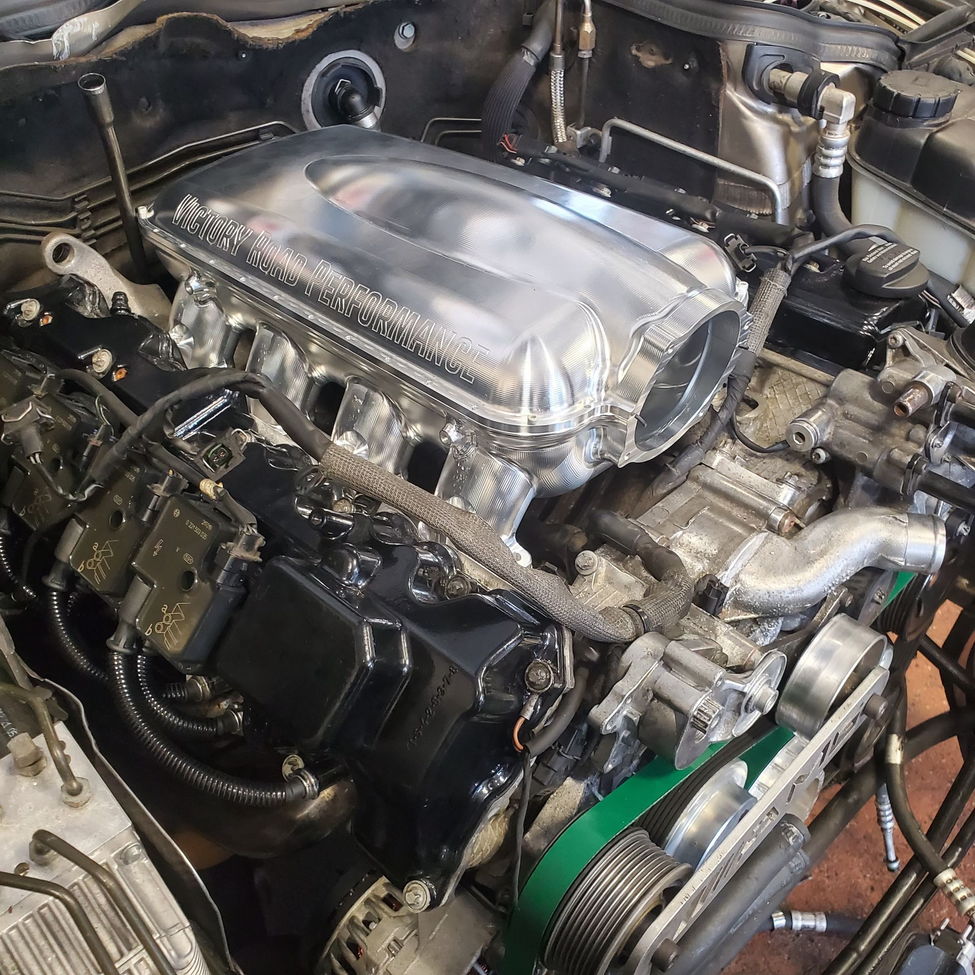This color photograph showcases the intricately detailed and metallic interior of a car engine with the hood open. Dominating the scene is a large and shiny supercharger on top, with "Victory Road Performance" engraved on it. Surrounding the supercharger are multiple chrome parts, adding to the pristine and clean appearance of the engine. To the left side of the supercharger is a sizable black component, possibly a fluid reservoir for the windshield. The lower part of the engine features a distinctively green belt, presumably the only colorful element amidst the metallic and black hues. The green belt, which appears slightly misaligned, could be the fan or timing belt. The right side of the engine is replete with tubes and hoses, while the back end, near the passenger compartment, is also visible in the background.